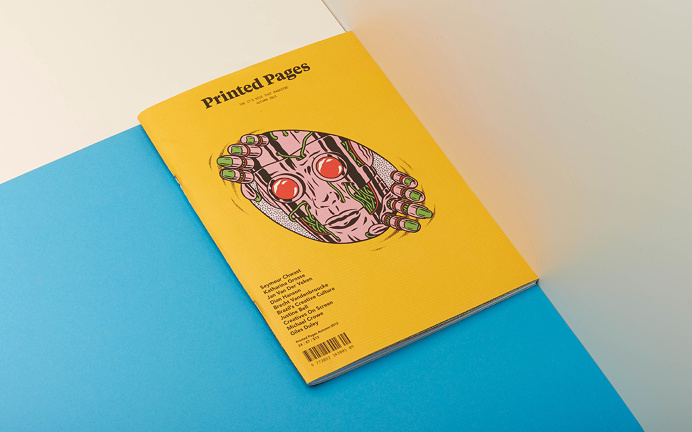The image features a yellow book titled "Printed Pages," prominently placed at the intersection where a blue sheet meets a white sheet, creating a dividing line between the two colors. The background also includes a silver-colored, wall-like object toward the right. The book's cover features a striking illustration of a mechanical, humanoid figure emerging through a circle. The robot-like figure's hands extend out of the circle, and it stares directly at the viewer with two large red eyes. Its mouth is depicted with visible wires. Additionally, the bottom left of the book cover contains a barcode and some text, possibly a list of names or related information.